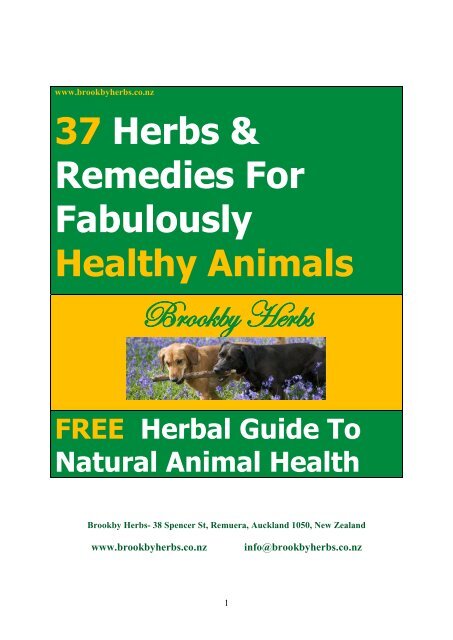This image is an advertisement for Brookby Herbs, featuring a green background with white and yellow text. Across the center, there is a yellow rectangle containing a picture of two larger dogs, a black lab and a light brown lab, each holding one end of a stick. They are standing in a field of green grass with purple flowers. The advertisement promotes "37 Herbs and Remedies for Fabulously Healthy Animals" and offers a "Free Herbal Guide to Natural Animal Health." The text includes multiple mentions of the website www.brookbyherbs.co.nz and contact information including Brookby Herbs, 38 Spencer Street, Remuera, Auckland, 1050, New Zealand, and email info@brookbyherbs.co.nz.